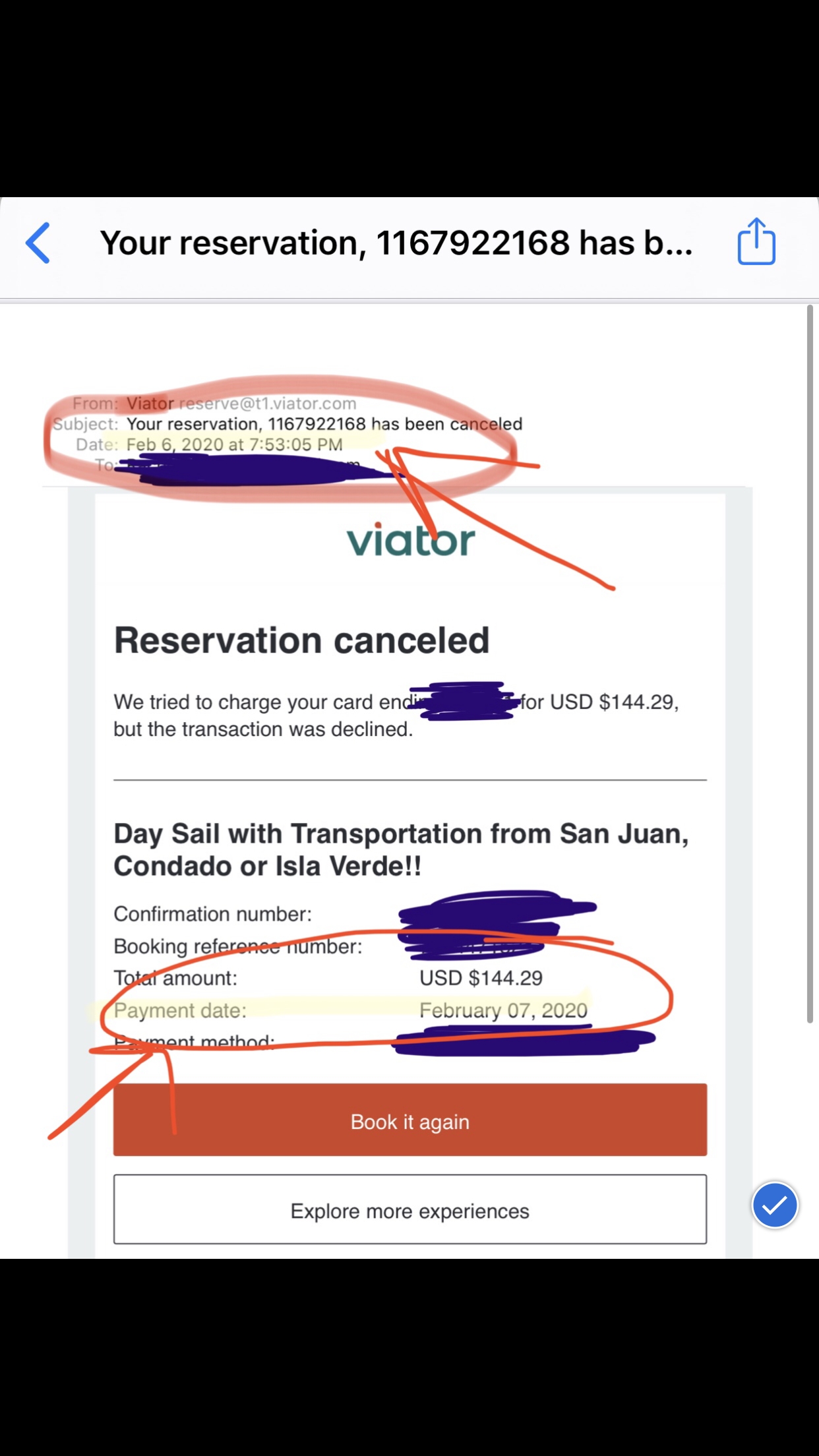In the image, there is a screenshot displaying a reservation cancellation notification. The page announces that reservation number 1167922168 has been canceled. The cancellation occurred on February 6th, 2020, at precisely 07:30:05 PM, originating from vieto.reserve at t1.vieta.com. The notification explains that the reservation was canceled because an attempt to charge the card ending with (specific digits not shown) for the amount of USD $144.29 was declined.

The reservation entailed transportation services from locations such as San Juan, Condado, or Isla Verde. Due to privacy, both the confirmation number and the booking reference number have been obscured or not shown. Users are prompted to rebook the reservation, with the total cost mentioned as USD $144.29. 

The image itself is framed with black bars at both the top and bottom, suggesting it might have been captured or cropped from a widescreen device.